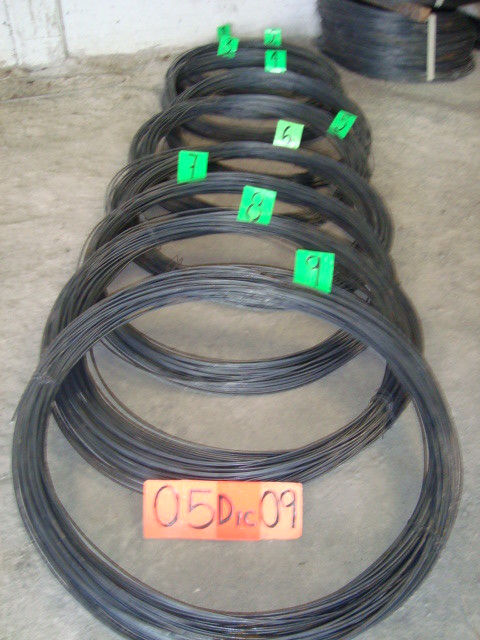In a room with white concrete walls and a light gray, sandy-textured floor, nine coiled bundles of dark gray or black plastic-coated electrical wires are neatly displayed in a cascading line from the foreground to the back center of the image. Each coil is tied and tagged with a green label numbered sequentially from 1 at the far end to 9 at the closest end. In front of the second bundle lies a yellow-orange tag inscribed with the black text "05DIC09." Towards the upper right-hand corner of the image, a pile of additional wire coils can be seen resting on their sides. A partial view of a table leg extends over a larger coil of wires in the background, adding to the industrial setting.